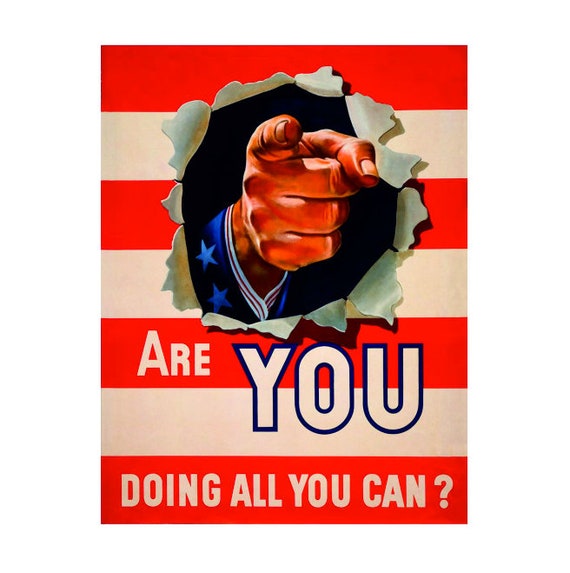The image is a vintage military recruitment poster with a stark white background. Dominating the center, it features a hand bursting through a red and white striped flag, which looks as though it has been torn like paper to allow the hand to break through. The hand is garbed in a sleeve adorned with blue and white stars, evoking elements of the American flag. The stripes of the flag are red, white, red, white, red, white, and red, suggesting a patriotic theme. The text "ARE YOU DOING ALL YOU CAN?" appears in bold, uppercase letters on the red stripes, with the word "YOU" emphasized in white against a blue border. The dimensions of the rectangular poster are such that the height is half the width. The overall message of the poster is a call to action, reminiscent of traditional Uncle Sam recruitment posters but with a reversed focus, asking the viewer if they are contributing as much as they can.